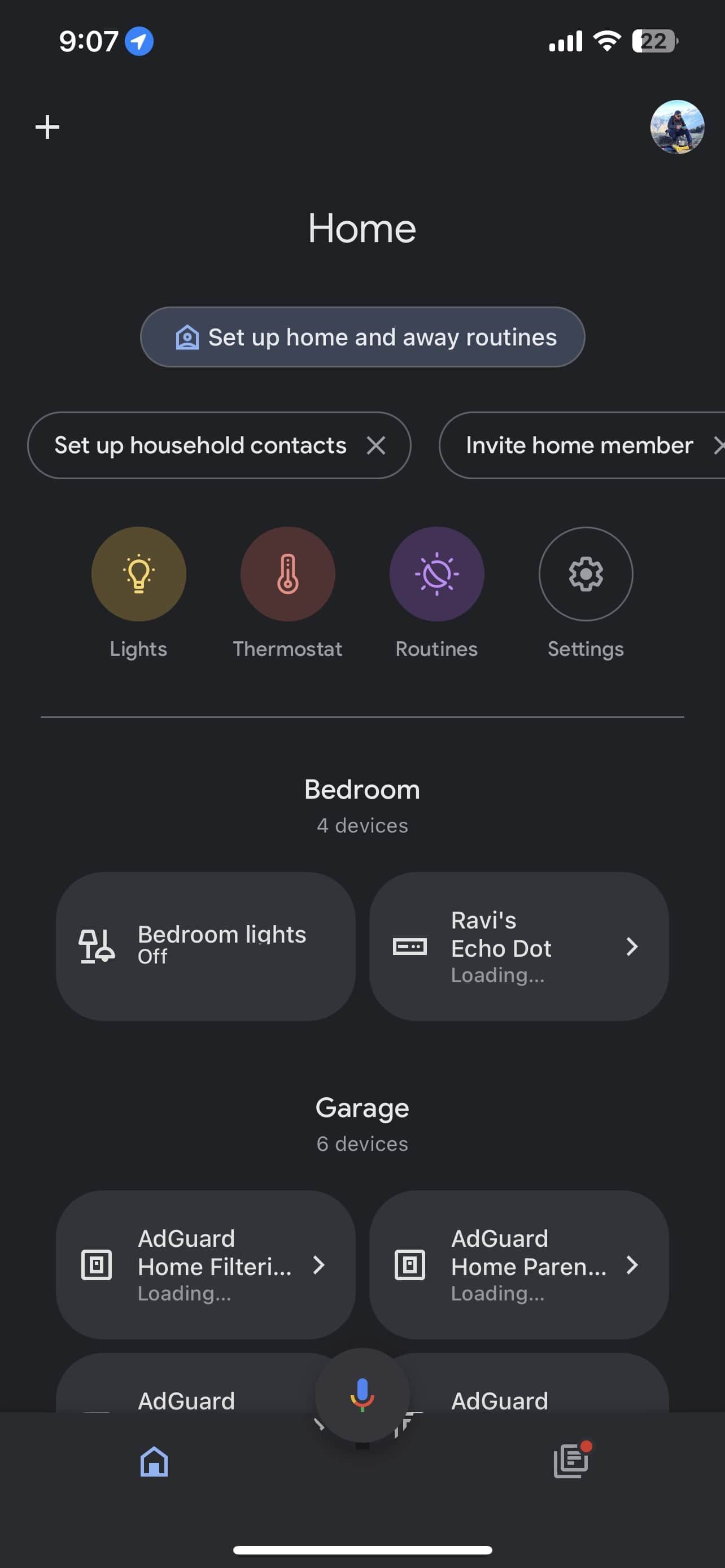Here's a detailed and cleaned-up descriptive caption for the image of the mobile real estate website:

---

The image showcases a mobile real estate website interface. At the top of the interface, the header prominently displays the word "Home" in the center. Directly below this header, there are three distinct bubbles. The first bubble reads "Set up home and away routines." Beneath this primary bubble, there are two additional bubbles. The one on the left instructs users to "Set up household contacts," while the one on the right prompts to "Invite home members."

Further below, there are four icons representing different functionalities within the home system. The first icon, depicting a light bulb with a yellow background, is labeled "Lights." The second icon, a thermostat with a red background, is labeled "Thermostat." The third icon, resembling a clock dial with a purple background, is for "Routines." The fourth icon is a gear, representing "Settings."

In the subsequent section, the interface categorizes different parts of the home. The first category is "Bedrooms," which includes four devices. The first two devices listed are "Bedroom lights off" and "Ravi's Echo Dot." 

The next category is "Garage," showcasing six devices, with the visible ones being "AdGuard Home Filtering," "AdGuard Home Parenting," and two other sections related to AdGuard.

At the bottom of the interface, there's a black footer featuring a microphone icon in the center for voice interactions. The footer also has two icons: on the left side is a blue house icon, and on the right side, there is a stack of papers with a red dot at the corner, indicating notifications or alerts.

---

This caption provides a comprehensive and structured description of the mobile real estate website interface.